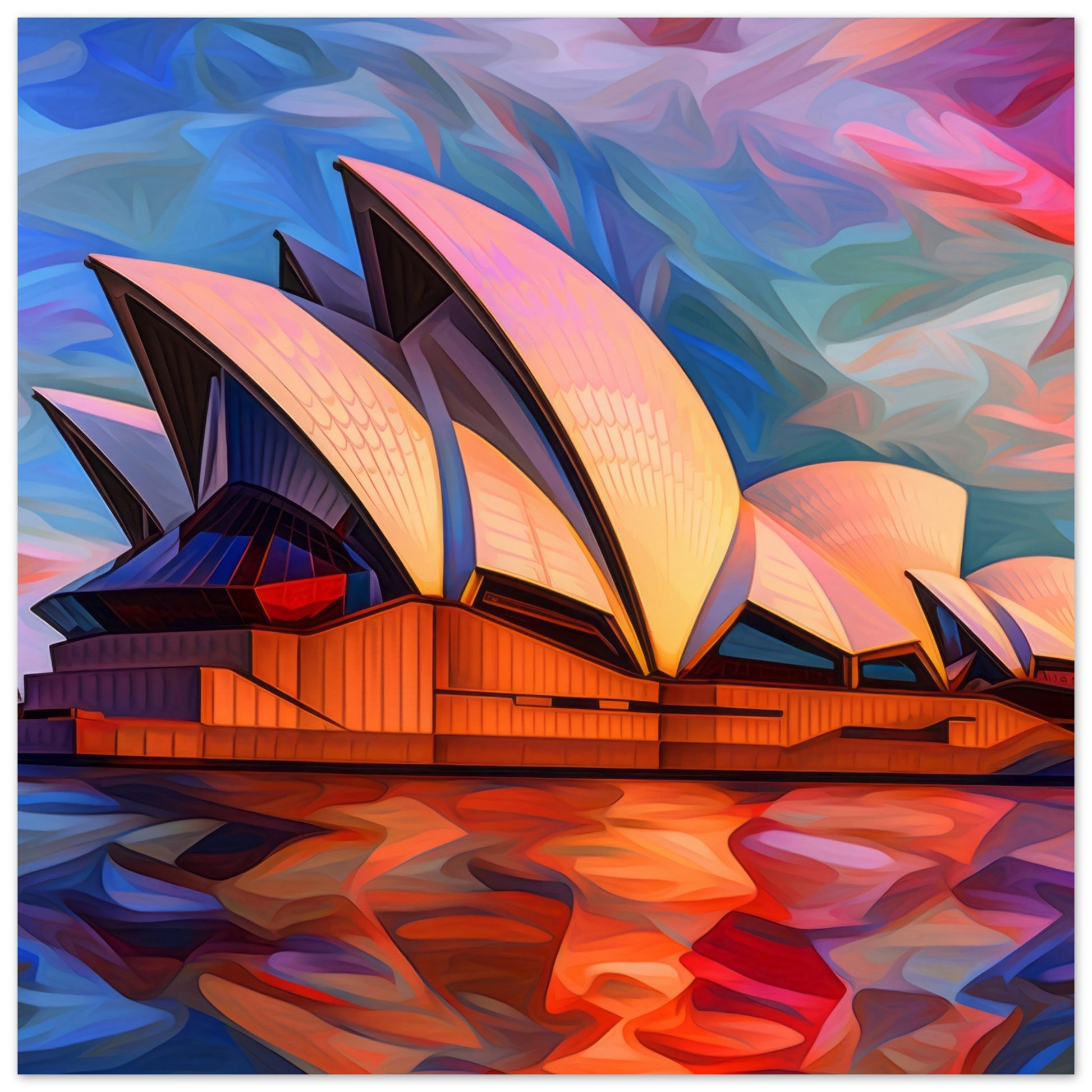This painting of the iconic Sydney Opera House in Sydney, Australia, captures the landmark with artistic flair. The base of the building features a wooden or brown hue, from which geometrically intriguing windows extend. Atop the structure, there are striking white arcs reminiscent of seashells or sailboat sails, adding a futuristic touch. The sky and water are depicted in an impressionistic, abstract manner, blending a rich palette of colors: blues, pinks, purples, and greens. The water vividly reflects the building, incorporating oranges and darker shades, while the sky transitions from blue and pink to violet and cyan, infused with light greens. The overall composition conveys both the grandeur of the Sydney Opera House and the dynamic, colorful essence of its surroundings.